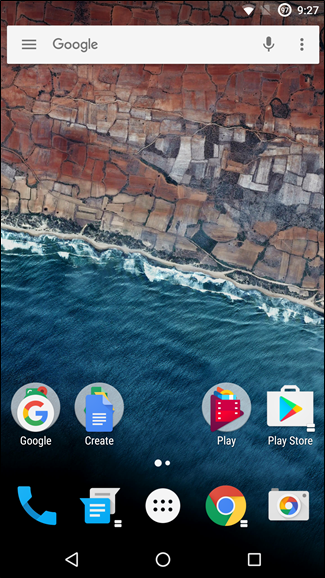This is a detailed caption of a digital image captured as a phone screenshot. The background scenery showcases an expansive ocean with small waves gently undulating on the surface. Prominently featured are majestic red, yellow, and white rock formations that form an intriguing cave-like structure. The time displayed on the phone is 9:27. At the top of the screen, a Google search bar is present, complete with a small microphone icon, three vertical dots, and three horizontal lines for additional options. Displayed below are various app icons. The recognizable Google app icon is seen, followed by an app labeled "Create." The Play Store app icon is also visible, characterized by a briefcase symbol and a sideways triangle with a palette of blue, green, red, and yellow colors. The screen includes a blue phone icon, a blue and white messaging icon, and the distinct Google Chrome icon, which features concentric circles in red, green, and yellow with a central blue dot.